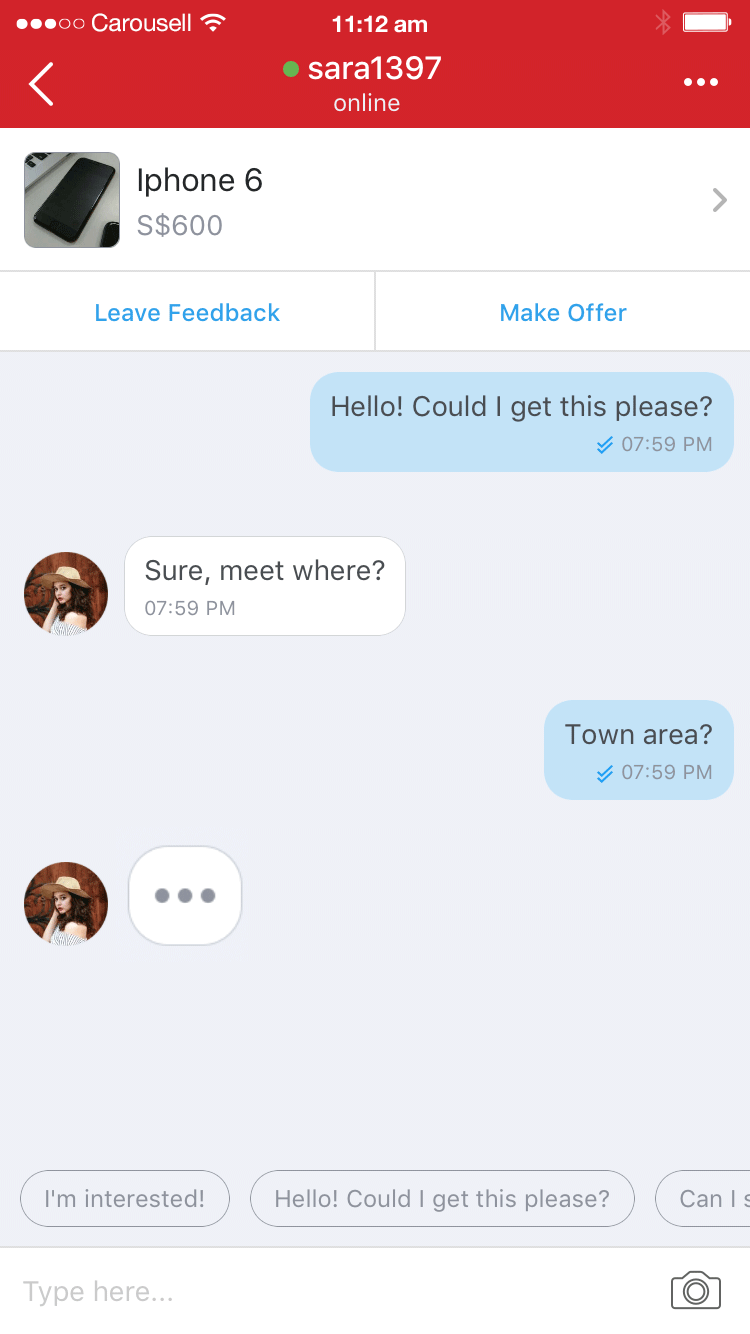Screenshot of a conversation displaying a buyer's request to purchase an iPhone 6 for $600 from an online marketplace. In the chat, the interested buyer initiates the conversation at 7:59 PM, asking, "Hello, could I get this please?" The seller promptly replies, "Well sure, meet where?" The buyer suggests meeting in "town area," while the seller's response shows as three typing dots, indicating they are in the process of drafting a reply. This screenshot captures the moment just before the seller specifies the meeting location, depicting the ongoing negotiation of the meeting place for the exchange.